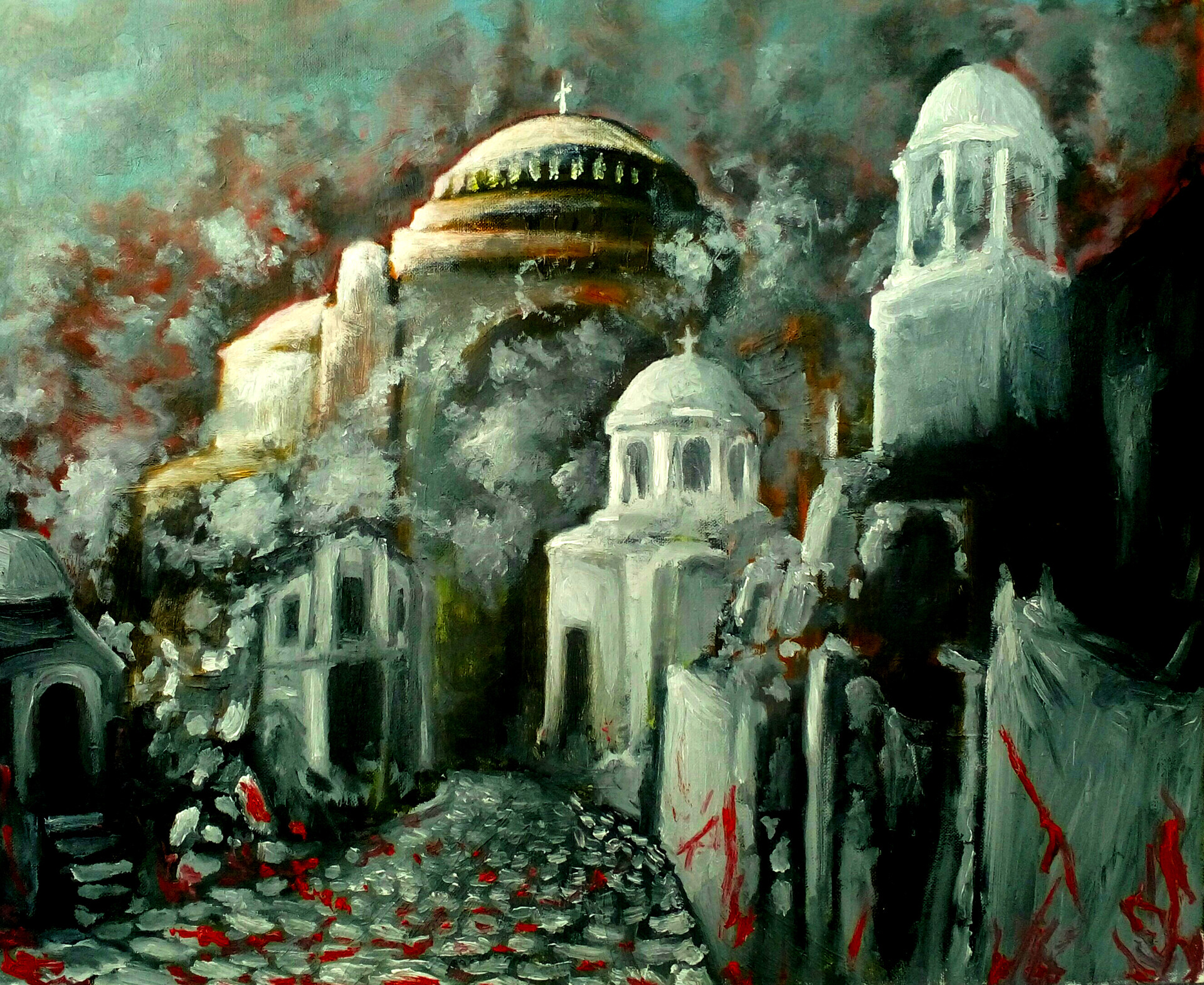The painting depicts a scene that seems to be set in a historical European city, possibly Rome given the architectural style. At the center top of the artwork is a prominent church with a small white cross perched atop a shallow dome. The church, partially obscured by white splotches and hazy elements, conveys a sense of age and wear. To the right and slightly below this central building, there's another dome-topped structure featuring an open area with arches and a small cross. Adjacent to this is a taller building with pillared architecture. The foreground of the painting reveals a gray stone pathway interspersed with darker hues, reminiscent of an old European roadway. Some areas, especially along the walkway and on certain building walls, are marked by streaks and red splotches, giving an impression of chaos or perhaps a historical battle scene. The background contains clouds tinted with gray and red, enhancing the tumultuous atmosphere. Additionally, red-colored trees add to the dramatic effect of the setting. Overall, the presence of multiple crosses suggests a religious significance to the scene.